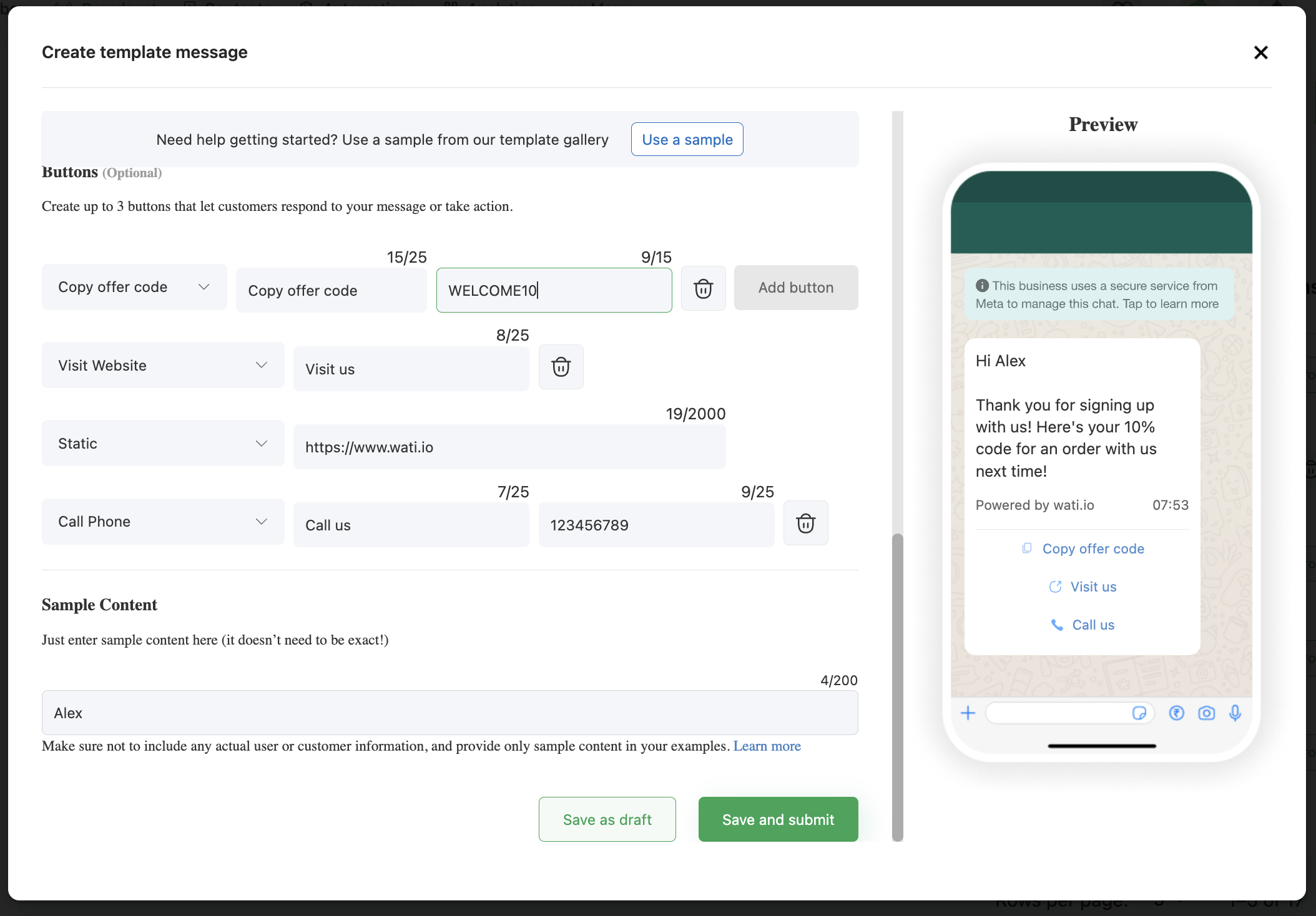In this image, the user interface for creating a template is displayed prominently against a white background. At the top left of the page, the heading "Create a Template Message" is visible. Directly below this, a suggestion is provided: "Need help getting started? Use a sample from our templates gallery," accompanied by a blue button labeled "Use a Sample."

The central section of the page includes several fields and buttons for customizing the template. There are three main buttons intended for customer actions:
1. "Copy Offer Code" - Allows customers to copy a promotional code.
2. "Visit Website" - Redirects users to the URL "wati.io."
3. "Call Us" - Provides a space for entering a contact number.

Additionally, there's a section labeled "Create out of three buttons that lets customers respond to your messages or take action," highlighting the interactive elements available for customization.

Further down, there’s a sample content input field with a placeholder text: "Just enter a sample content here. It doesn't need to be exact." The example text entered here is "Alex." Beneath this input, a cautionary note advises, "Make sure not to include actual user or customer information and provide only sample content in your example."

Two options are available at the bottom for saving the template:
1. "Service Draft" - Displayed in green text but not filled.
2. "Service Submit" - Filled with green color, indicating the option to submit the template.

To the left side of the screen is a preview area simulating a smartphone display. At the top of the preview, a message states, "This business uses a secure service from Mesa to manage these chats." Below this, a text block reads: "Hi Alex, thank you for signing up with us. Here's a 10% code for another order with us next time. Powered by wati.io 753." The three actionable buttons—"Copy Offer Code," "Visit Us," and "Call Us"—are also depicted here, shown in blue, consistent with their customizable nature.

This comprehensive interface allows users to craft and preview customer interaction templates effectively.